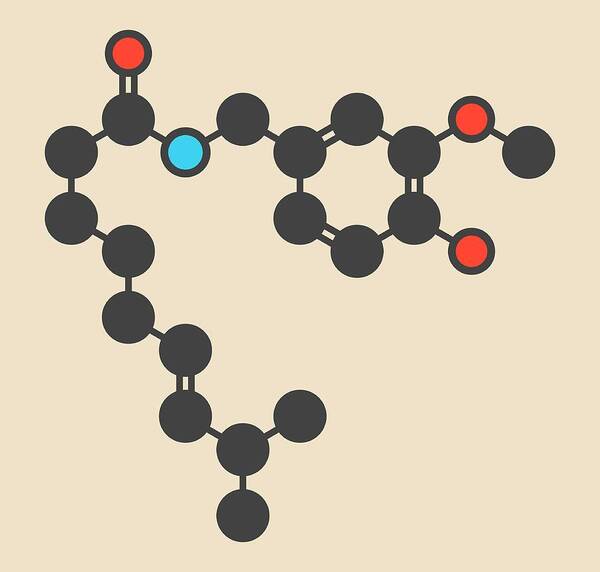The image features a piece of shape artwork on a cream or beige background, resembling a molecular diagram. It showcases 20 circles interconnected by either one or two lines, mimicking chemical bonds. The majority of the circles are a chocolate brown or black color. Interspersed among them are three orange-filled circles outlined in dark brown and one distinct blue circle, also outlined in brown. These circles form a complex structure that begins at the bottom center, curving upwards to the top left before taking a right turn across the top portion of the image. At the center top, six circles are connected to create a hexagonal loop. This intricate network of circles and lines suggests a visual representation of a molecular structure, with the colored circles highlighting potentially significant variations within the pattern.